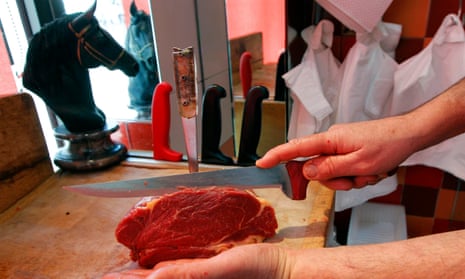In this detailed image, a man is meticulously slicing a large, red slab of meat on a light wooden cutting board. The scene is framed by his two hands: one gripping a long, sharp silver-bladed knife with a dark red handle, and the other steadying the meat from the left. The photograph captures the precise moment of the cut, with both hands and part of the arms visible, while the rest of his body is cropped out of the image.

In the background, there is a variety of elements adding to the depth and context of the setting. On the left side, a black horse's head figurine stands prominently, likely acting as a decorative piece. Adjacent to it, the reflective surfaces of mirror panels flank a white door, creating an impression of additional space. To the right, rows of white plastic bags hang neatly, suggesting a utilitarian purpose, possibly for bagging the meat. Below them, the knife handles of various colors—red, black, and wooden—are visible, sticking out from a slot at the end of the wooden table. Additionally, the wall behind features a checkerboard-like tile pattern, adding a structured backdrop to the busy scene.